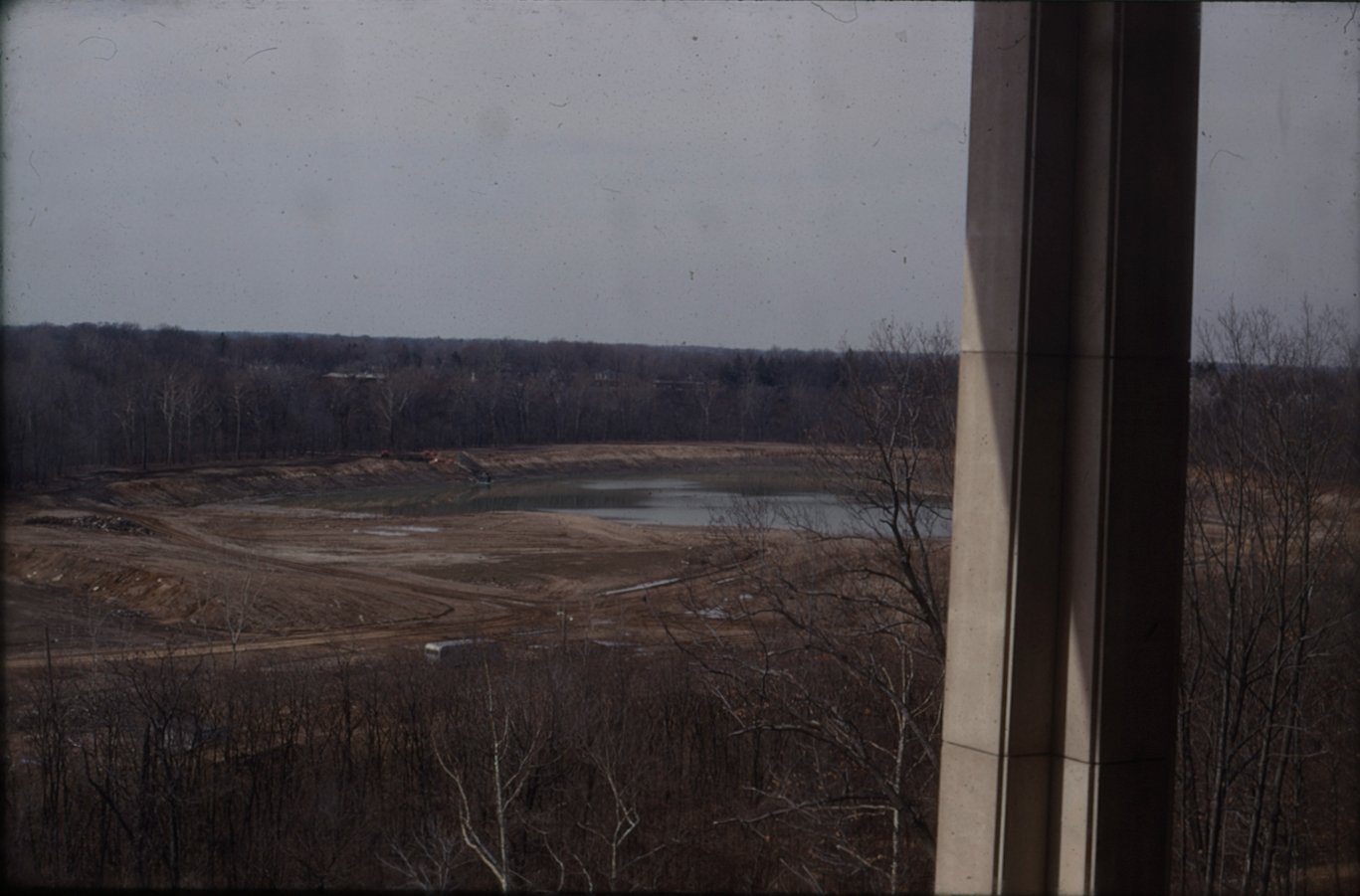This photograph, seemingly taken through a window or screen, captures a dreary, overcast scene centered around a barren landscape surrounding a large, dirty brown body of water. On the right side of the image, a prominent grey stone pillar extends to the top of the frame, marked by horizontal lines that divide it into three parts. The pillar casts a shadow on its right side and upper part. The outdoor area depicted in the image features leafless trees, indicative of winter, encircling the water, which appears to be a cesspool. The land around the water is barren and devoid of grass, crisscrossed by dirt roads. Notably, a silver-colored bus or van is seen on one of the roads, enhancing the sense of abandonment and desolation. The sky above is grey and overcast, adding to the dark and dreary atmosphere of the scene.